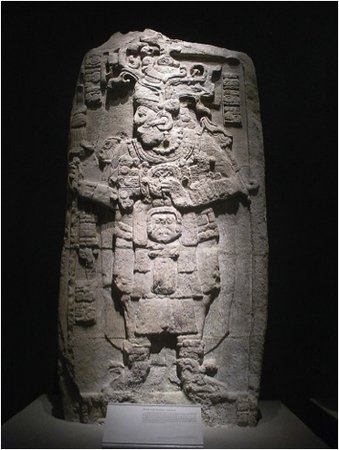This is a photograph of an ancient stone carving, possibly of Chinese origin, prominently displayed in a museum. The carving is a tall, cylindrical relic made of light gray stone, with a rough texture. It depicts a full-body profile of a man in elaborate attire, complete with detailed carvings of robes, headgear, and decorations on the garment. The man is oriented to the left, with his elbows pointed out and hands positioned in front of his chest. His feet are visible at the base of the carving.

The artifact rests on a light-colored platform, which may be stone or a similar material. The background is entirely black, enhancing the focus on the relic, with professional lighting casting a spotlight on the center, creating shadows around the edges. A white placard with black text, attached to the base, indicates that this piece is an important exhibit, though the text is illegible due to the photograph's resolution. The overall scene suggests that this is a highly valuable and well-preserved piece of historical art, meticulously highlighted in a dark museum environment.